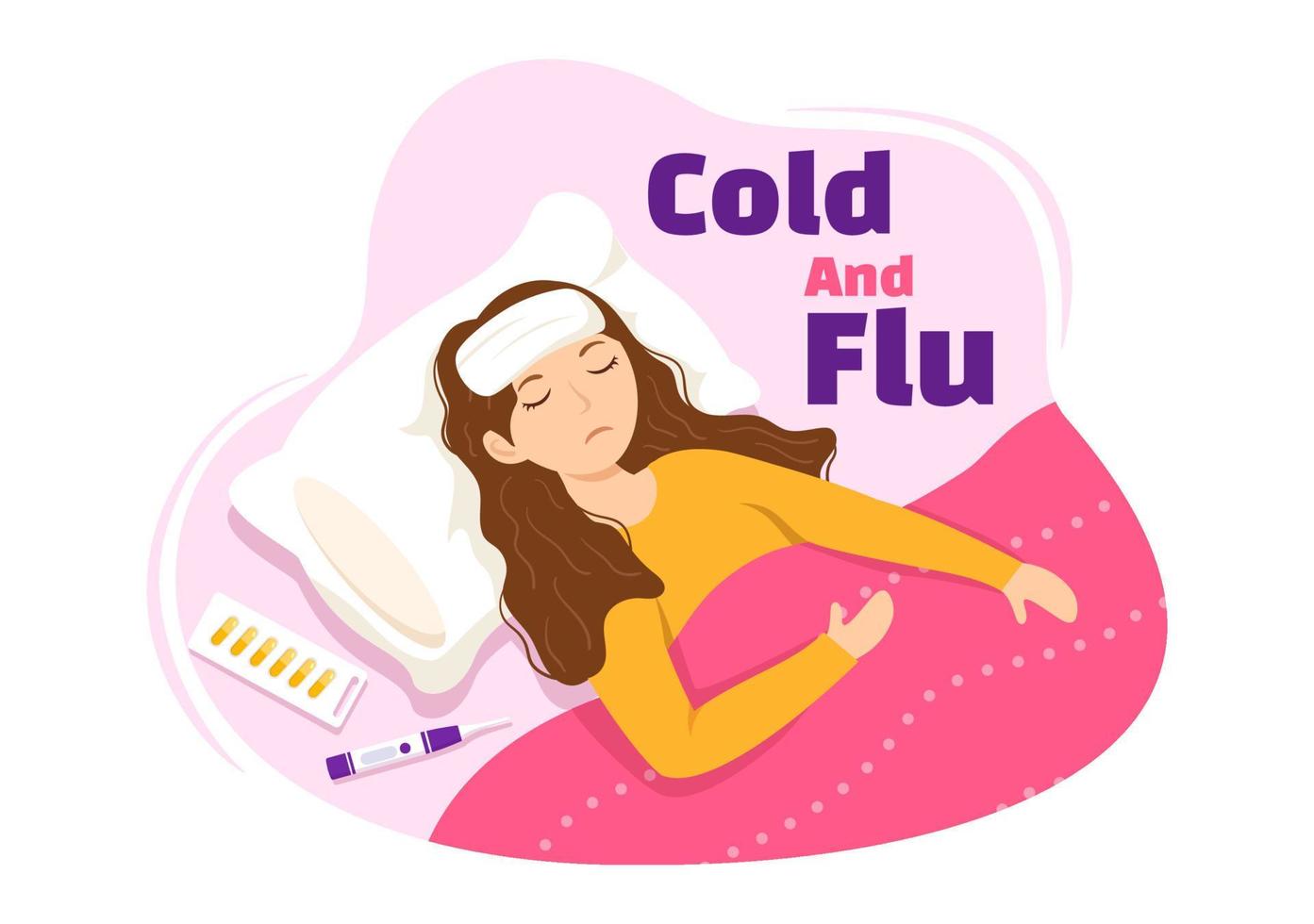The image is a detailed, animated graphic of a sick female laying in bed. She has long brown hair and her eyes are closed, suggesting illness. She has a white cold compress on her forehead and is wearing a long-sleeved yellow top, likely pajamas. She lies on a white pillow under pink covers with white dots arranged in two lines. Next to her is a thermometer with purple accents and a white tip. The border of the image is cloud-like, adding a cozy yet illustrative feel. There is a standout text in the image, where "cold" is written in capitalized red letters, and "flu" is in capitalized purple letters, emphasizing the theme of health and sickness. Her arm positioning indicates rest and recovery. Additional details include a case with yellow and orange accents near the pillow. This image appears to be an advertisement or informative graphic about cold and flu, illustrating the typical resting state and care methods during illness.